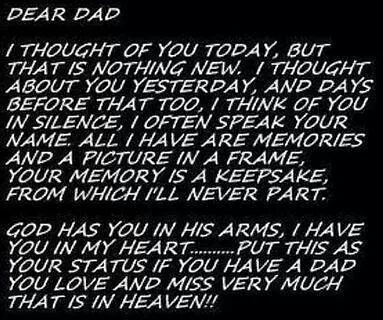The image is a small black square featuring a heartfelt message in bold white cursive text at a slight angle. The text reads, "Dear Dad, I thought of you today, but that is nothing new. I thought about you yesterday and days before that too. I think of you in silence. I often speak your name. All I have are memories and a picture in a frame. Your memory is a keepsake from which I'll never part." Below this, another line in the same white cursive text says, "God has you in his arms. I have you in my heart...... Put this as your status if you have a dad you love and miss very much that is in heaven!!" The black background and white text create a stark contrast, making the poignant message stand out. This image appears to be a sentimental status update shared on social media, reflecting on the enduring love and memories of a father who has passed away.